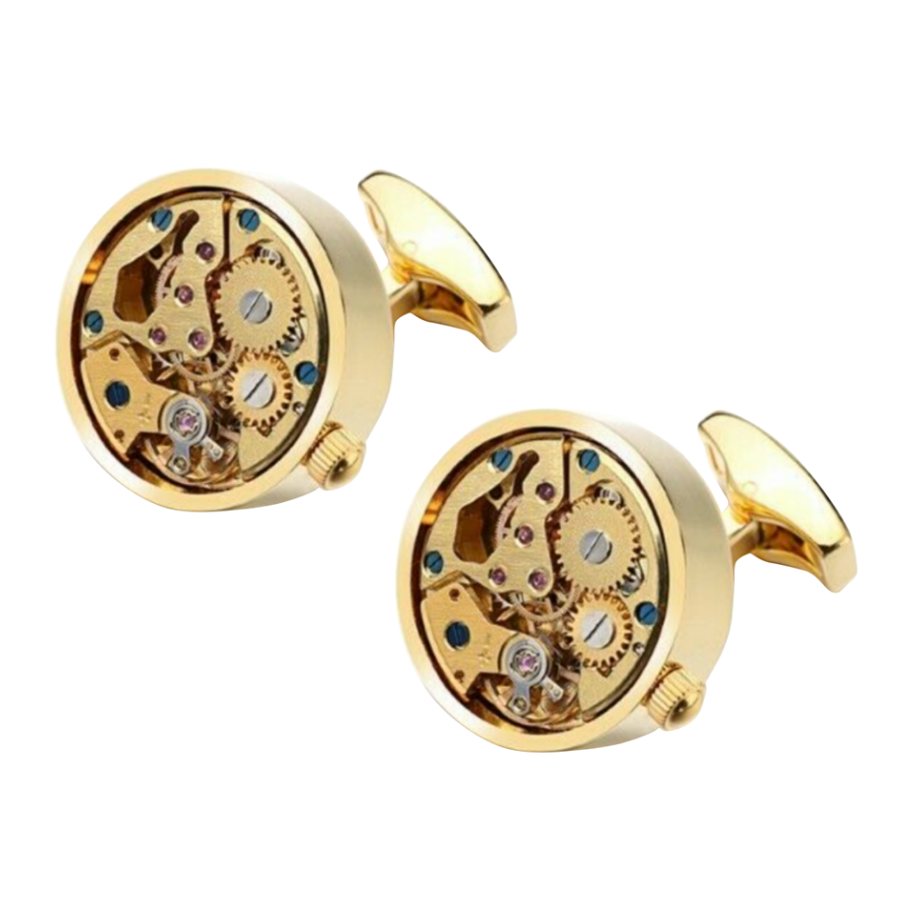This photograph captures two identical, high-quality gold cufflinks designed to resemble the intricate interiors of watches. Each cufflink features exposed gears, with the gears and other components meticulously detailed in gold. The screws within are a striking blue-black, some silver, and copper, adding a dynamic contrast to the gold elements. The cufflinks are arranged diagonally with one in the top left and the other in the bottom right, all set against a clean, white background that emphasizes the luxurious shine and detailed craftsmanship of the pieces. The back of each cufflink is folded out, revealing polished, rectangular-shaped gold bars designed to secure through a buttonhole. Despite their remarkable simulation of timepiece mechanics, including winding stems and potentially even a jewel, these cufflinks are stationary, designed purely for aesthetic elegance. The perfect lighting in the photograph highlights the brilliance and pristine condition of the cufflinks, showcasing them as sophisticated accessories rather than functional timekeepers.